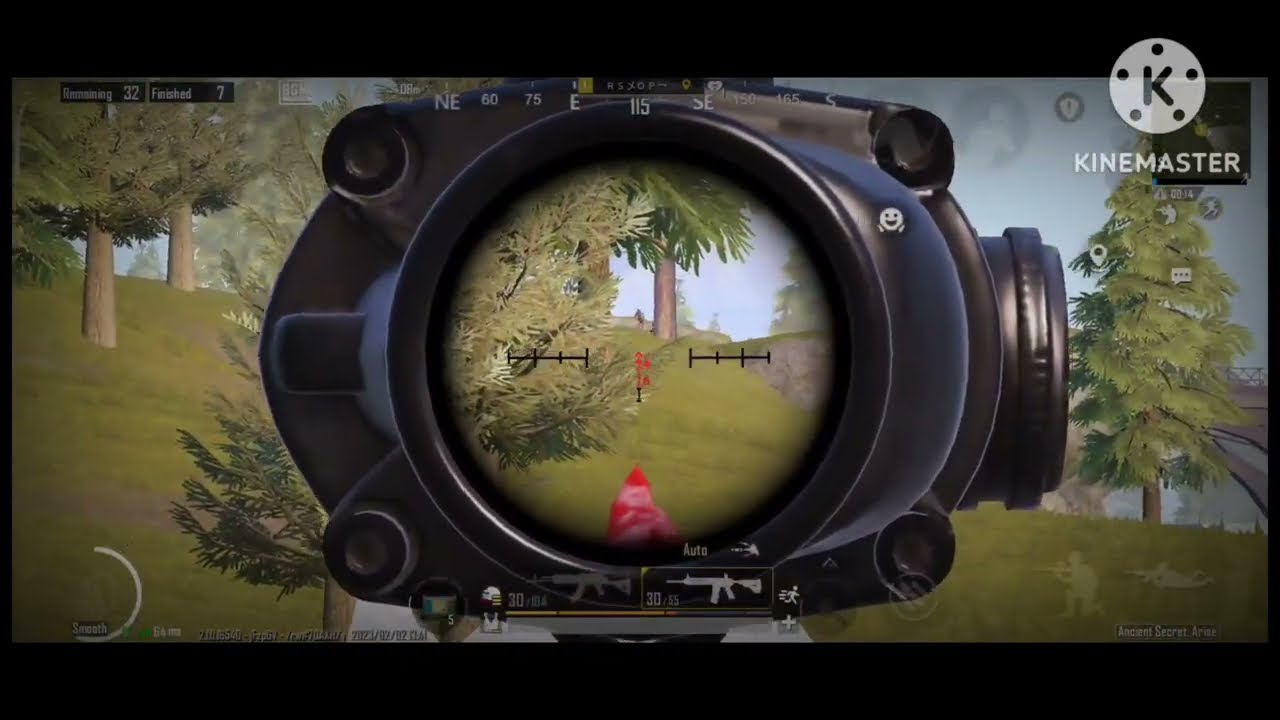In this detailed screenshot of a first-person video game, we see a scene framed as if viewed through a single lens, possibly simulating a scope or binoculars. The foreground is dominated by vibrant, green grassy hills and tall, green trees, with a distinct red figure standing in the middle of the landscape. This red figure is targeted by a large bullseye, giving the impression that the player is aiming at it, potentially preparing to shoot. The bullseye appears to be part of a sophisticated aiming system, perhaps attached to a gun, microscope, or magnifying lens.

At the top right corner of the screen, "KineMaster" is prominently displayed, accompanied by a round white logo featuring a black letter "K" surrounded by black dots. The upper left corner indicates "remaining 32 finished 7," suggesting gameplay statistics. The background reveals a grey sky amidst a forested environment filled with bushy trees and dense foliage.

In the bottom right corner, faint images of two soldiers can be discerned: one lying on the ground with a weapon, and the other kneeling with his weapon at the ready. Additionally, a unique smiley face is subtly integrated into the camera lens interface. Overlaying the top of the screen, the vision range is noted, fluctuating between 65, 75, 90, and 115, reinforcing the immersive nature of the gameplay.